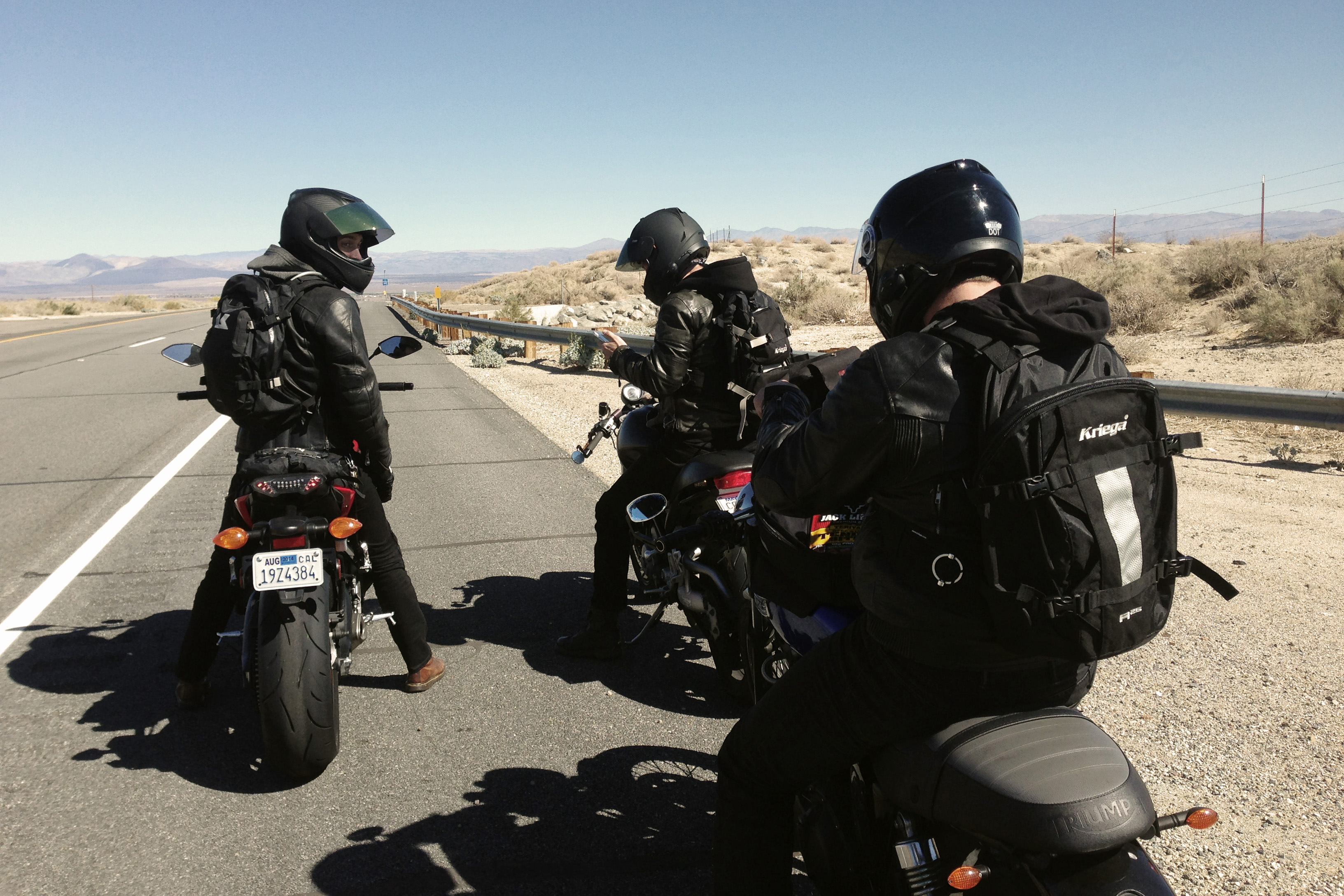The photograph captures a trio of motorcyclists stopped on the shoulder of a wide-open desert highway. All three riders are clad in black helmets, black leather jackets, and black backpacks, seated on black motorcycles, each of a different style. One of the motorcycles, identifiable by the "Triumph" written on its seat, stands out among the group. They're positioned on the right side of the road, which features a gravelly, dirt shoulder and a metal railing. The arid landscape around them is dotted with scrubby bushes and low-lying green scrub, stretching out into the distance. Telephone or electrical lines run alongside the road, leading the eye toward a hazy mountain range under a clear, cloudless sky that gradients from light to deeper blue. The road itself includes a solid white line on the left edge and a broken white line dividing two lanes, mirroring the barren, scrub-covered terrain on the other side.